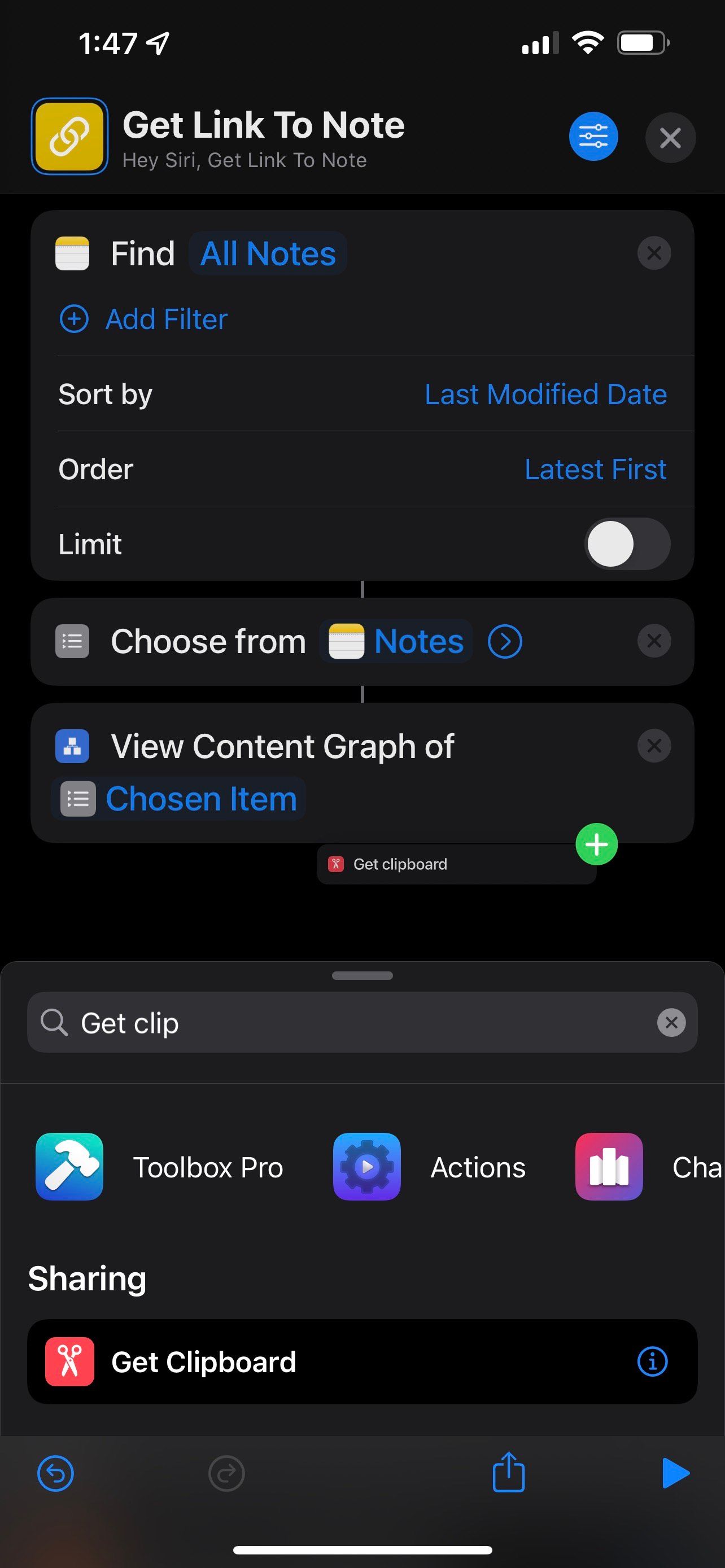The image appears to be a screenshot of a digital interface, possibly related to an Apple Store or a productivity application. The top left corner displays the time as "1:47" in white text, accompanied by a location arrow pointing slightly upwards to the right. Next to it, there are four signal bars, three of which are filled, indicating a strong network connection. To the right of the signal bars, there is a full Wi-Fi symbol, and further to the right, a battery icon shows approximately 80% charge.

In the bottom left corner, there's a yellow icon with three interlocking chain links and the text "Get link to note" in gold, accompanied by smaller white text below that reads, "Hey Siri, get link to note." Moving to the right, there is a blue icon featuring three horizontal slider bars, and next to it, an 'X' symbol. Below these icons, the text "Find all notes" appears in blue, followed by "Add filter" with a blue plus sign to its left. Further down, the text "Sort by" appears, with "Last modified date" listed to the right, followed by "Order latest first limit."

The top background of the image is black, transitioning to a gray screen further down. At the very bottom, there is a search bar and various icons. To the far left, a blue icon labeled "Toolbox Pro" with a hammer inside is shown. To its right, there is a purple gear icon labeled "Actions" in white text, and next to it, a purple bar graph icon with three ascending bars. Below these icons, the text "Sharing" is visible, next to a red icon featuring scissors and the text "Get clip."

This detailed layout suggests an interface designed for note-taking, organizing, and possibly sharing content, with various features tailored for user accessibility and functionality.